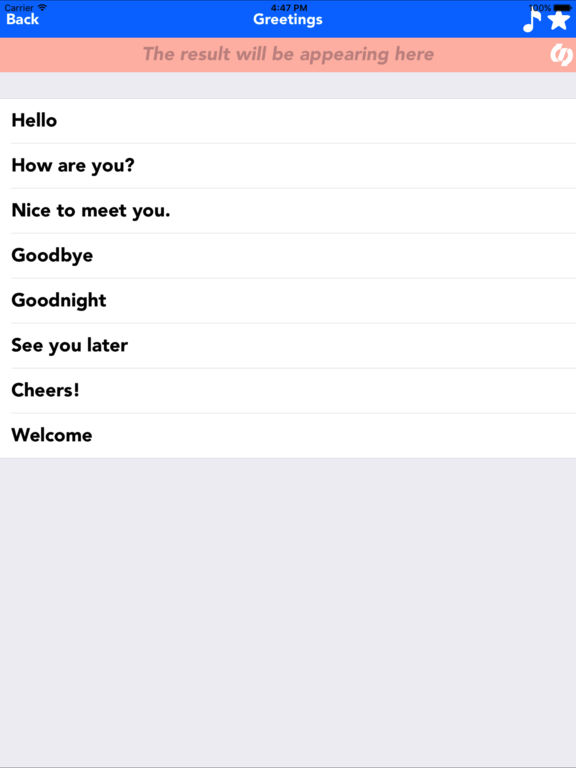This image is a vertically-oriented screenshot of a digital interface. At the very top, a blue strip banner displays three items: "carrier" in small black font at the upper left-hand corner, "4:47 PM" centered in black font, and "100% battery" at the upper right-hand corner. Directly beneath this strip, there is a navigation bar with the text "Back" on the left-hand side and "Greetings" in the middle. On the right end of this bar are a musical note and a star icon positioned under the battery indicator.

Below the navigation bar lies an orange-pink banner with the central text "The result will be appearing here." On the right side of this banner is a small white icon. Following this is a thin gray banner with no text or icons, serving as a separator.

The subsequent section features a vertically ordered list in bold black font, containing the entries: "Hello," "How are you," "Nice to meet you," "Goodbye," "Goodnight," "See you later," "Cheers," and "Welcome."

The bottom portion of the image is dominated by a large, empty, very pale light gray box. Ending the image is a very thin line at the bottom, with no additional detail. The screenshot lacks a border in the upper two-thirds below the heading banner.